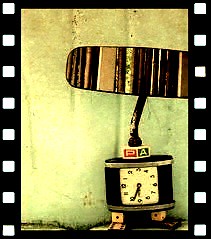In this vibrant image, the left and right edges are framed by black vertical lines adorned with white squares stretching from top to bottom. Horizontally across the top and bottom of the image are solid black lines without any squares, creating a distinct border. The background is primarily yellow, transitioning to a greenish hue as it approaches the ground, giving a gradient effect. At the bottom of the image are two white dice, each showing a single dot, indicating the number one. Poised atop these dice is a black object featuring a clock at its center. This clock has a white face with black numerals and hands, providing a stark contrast. Above the clock, there is a red square marked with the letter "P" and another square with the letter "A" in a darker hue. Extending from this setup is a pole, leading to a horizontally aligned skateboard-like shape at the top. This skateboard-like element incorporates vertical stripes in white, yellow, brown, and black, adding to the image's eclectic mix of shapes and colors.